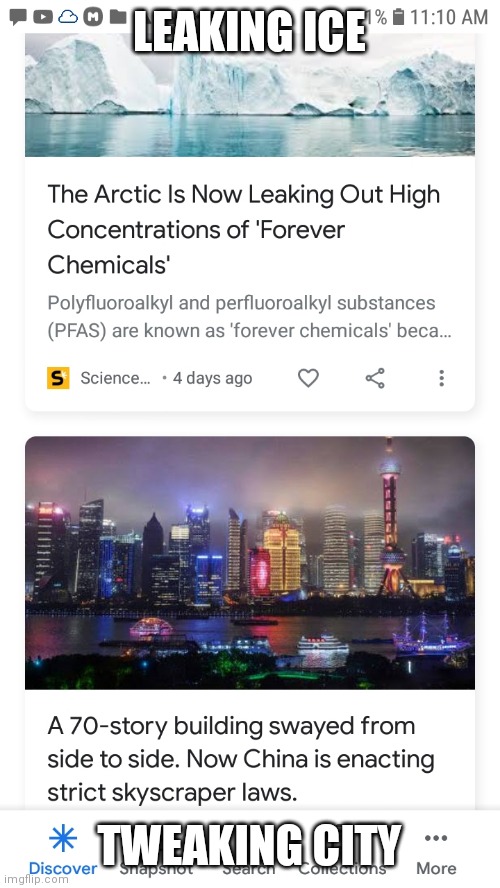This image appears to be a screenshot from an internet search or news website. At the top, there is a rectangular image showcasing serene, glass-like blue-green waters with icebergs in the background. Large white capital letters spell out "LEAKING ICE" across the top of this image. Just above it, the time is displayed as 11:10 AM. Beneath the headline are several small icons, often used for interactive features.

The article preview suggests that it is discussing the alarming phenomenon of high concentrations of polyfluoroalkyl and perfluoroalkyl substances (PFAS), also known as "forever chemicals," being released from the Arctic. However, only a portion of the text is visible, and it mentions that the information is sourced from a science magazine published four days ago. Below the preview, there are icons for liking, sharing, and additional options.

Adjacent to this, another article is headlined "TWEAKING CITY" and depicts a sprawling city skyline believed to be in China. The photograph captures numerous high-rise buildings along a waterfront during the evening, with a cloudy and hazy sky overhead. Several boats are visible on the water, illuminated by their lights. The caption references a recent event where a 70-story building swayed side to side, leading China to implement stricter skyscraper laws.